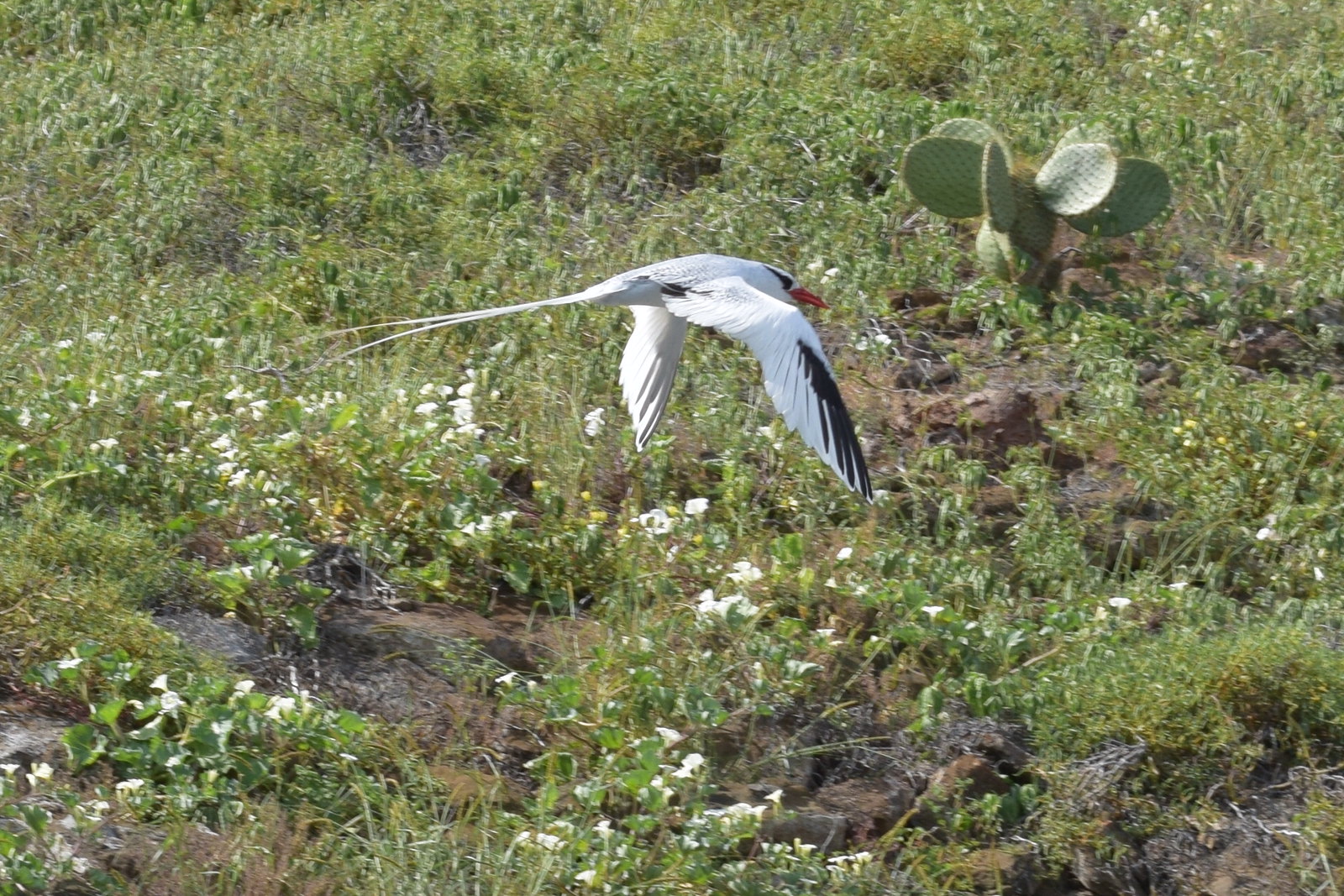In a verdant, fiery landscape filled with patches of blooming white flowers and scattered dirt, a magnificent bird flies from right to left. The bird, a striking creature never seen before by many, has primarily white plumage contrasted with black forewings, a black patch near its tail, and black above its eyes. It boasts a very dark orange bill and elegant, long pointed tail feathers with two distinctive stems protruding from its head. The ground below is adorned with rocks and greenery, including a prickly pear-shaped cactus to the right and various plants with green leafy wings. The scene lacks any signs of human development or structures, enhancing the natural beauty of the setting.